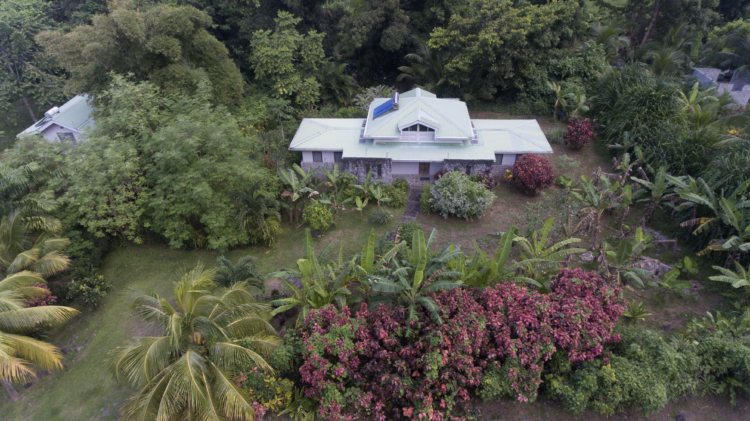This aerial photograph captures a lush, tropical scene with dense foliage that features three properties. The focal point is a two-story house centrally located within a verdant expanse. This house is distinctive with its white roof, beige walls, and solar panels positioned on the left side of the roof. A cobblestone porch and a small walkway lead to its entrance, adding to its charm. The house is surrounded by an array of greenery, including palm trees, various other trees, bushes with vibrant red flowers, and some floral bushes and trees in colors such as pink and yellow. On the left edge of the image, part of the roof of another building is visible, hinting at the presence of additional properties. The other two properties, one with a white roof and one with a gray roof, are nestled within the dense tropical vegetation, making their details less prominent compared to the central house. Grass and other lush vegetation dominate the scene, emphasizing the natural, tropical setting of this aerial view.